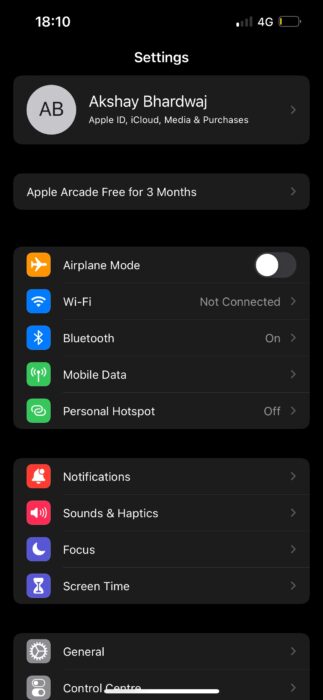Here's a detailed and cleaned-up caption for the image:

---

This image is a screenshot taken from a smartphone. At the very top, the status bar displays the time "18:10" in white text on the left. On the right side of the status bar, there are icons indicating a cellular signal, a 4G Wi-Fi connection, and a battery icon with a small yellow portion, suggesting low battery. Below the status bar, the screen shows the "Settings" menu, with "Settings" written in bold white letters and the "S" capitalized.

Directly beneath the "Settings" heading, there is a black banner featuring a gray circle with the initials "AB" in uppercase letters. Next to the circle is the name "Akshay Bhardwaj," written with a capital "A" and "B." Below his name, it reads "Apple ID, iCloud, Media & Purchases."

Further down, another black banner advertises "Apple Arcade" which is available "free for three months." The list of settings options follows, displayed in white text on a black background. The options include "Airplane Mode" (with a small circular icon indicating it is off), "Wi-Fi" (marked as not connected), "Bluetooth," "Mobile Data," "Personal Hotspot," "Notifications," "Sounds & Haptics," "Focus," "Screen Time," "General," and "Control Center."

At the very bottom of the screen, a thin white line is visible, indicating the navigation bar typical of modern smartphones. The entire background of the settings menu is consistently black.